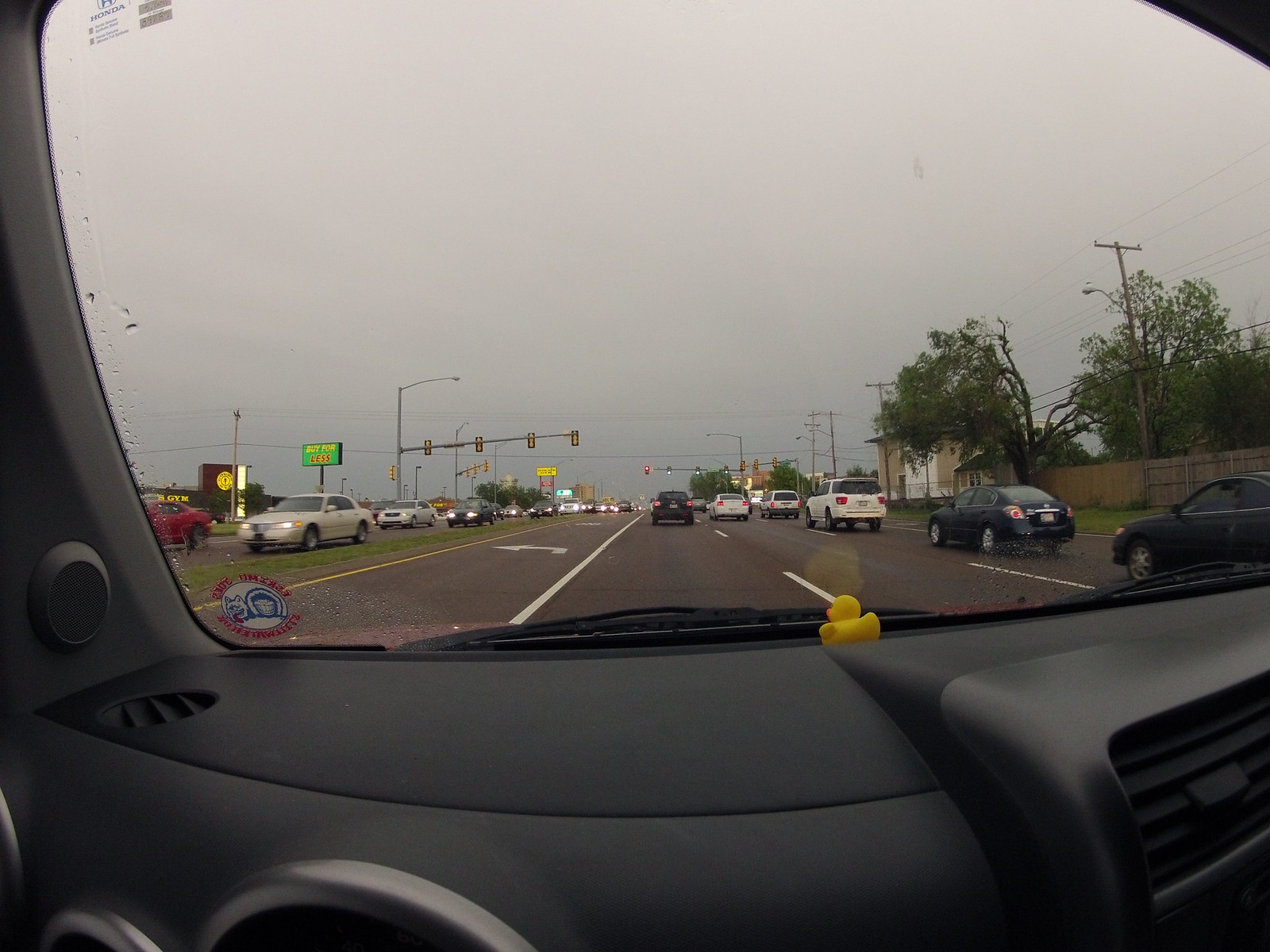A cloudy day sets the scene in this image, captured from the interior of a moving car. The black dashboard is prominently visible, featuring a whimsical yellow rubber duck right up against the windshield. Raindrops speckle the sides of the windshield, hinting at recent or impending rainfall. The car is traveling forward on a three-lane highway, plus an additional left turn lane. 

The traffic light ahead glows green, allowing several cars to proceed. Notably, the left turn lane is mostly empty, except for one car poised at the front, awaiting a signal change. To the right, two more lanes are visible, bordered by a stretch of grass, trees, a wooden fence, and telephone poles strung with wires. On the opposite side, beyond a grassy median, cars travel in the opposite direction. Further to the left, a strip mall housing various businesses appears to be coming into view.